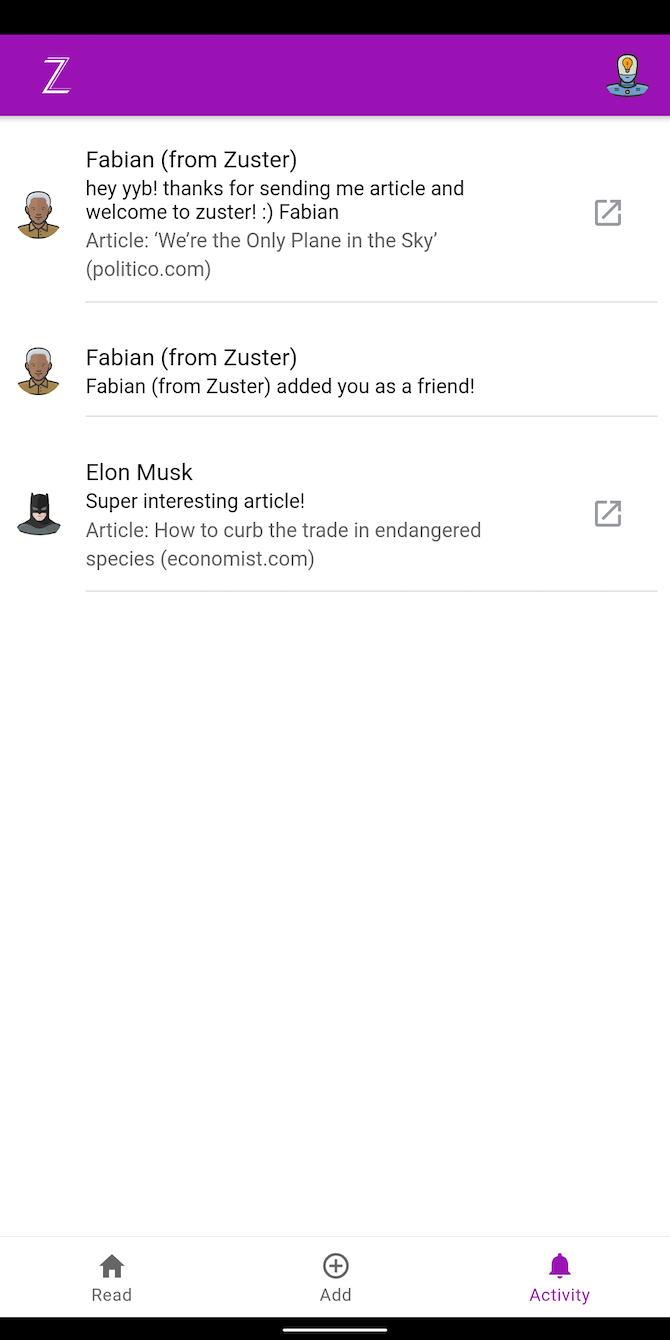This webpage features a series of distinct visual and textual elements, displayed in a somewhat complex layout. At the very top, there's a thin black banner, and directly beneath it spans a prominent purple banner stretching across the width of the page. On the purple banner's left side, a white "Z" is prominently visible, while the right side features an ambiguous image that somewhat resembles a hat.

Below these banners, the page contains three different articles. The first article on the left displays the face of a man, presumably named Fabian, and includes a brief description spanning three or four sentences. To the immediate right of this article, there is a small gray rectangle with a white background, featuring an arrow pointing either left or right. Directly beneath this, another similar gray rectangle is present.

On the next row, there is another image of a man’s head, possibly related to Fabian again, accompanied by additional textual content. Below this, on the left side, there appears to be an image of a hat—perhaps something related to Batman. To the right of this image, another article mentions Elon Musk and provides related information, completing the elongated and intricate layout of the webpage.